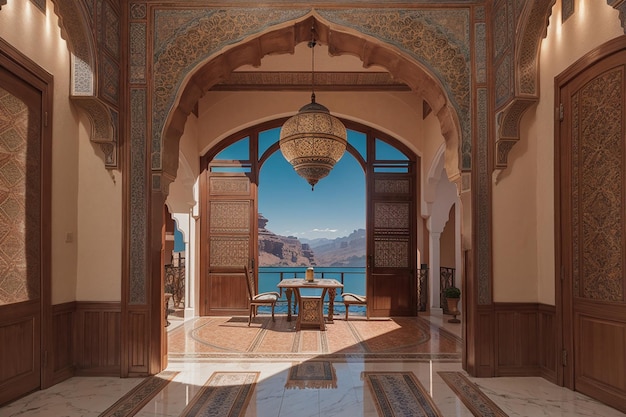The image depicts a luxurious room, reminiscent of a historical era, potentially from a vacation rental or hotel website. The foreground showcases a polished, reflective marble floor with rug detailing and predominantly earth-toned decor featuring browns, tans, and oranges. The walls are beige with intricate wooden designs along the bottom portion, and the archways, intricately carved and ornate, seamlessly connect the rooms.

The central archway, accented with delicate indentations and wood framing, leads to a secondary room with a table and two chairs. This room extends out to an elegant balcony framed by another ornate archway, offering a breathtaking view of a distant, brilliantly blue body of water, likely a lake, bordered by towering, orange-red rock structures or mountains. The balcony invites relaxation with its seating arrangement, ideal for soaking in the scenic landscape.

A notable feature in the second room is an exquisite, oval-shaped chandelier adorned with a woven structure, hanging majestically from the top of the arch. Additional subtle lighting elements are discreetly placed at the top left and right corners of the room. The exterior view through the archways not only reveals the stunning natural landscape but also includes a glimpse of the sky, enhancing the overall serene and elegant atmosphere of the space.